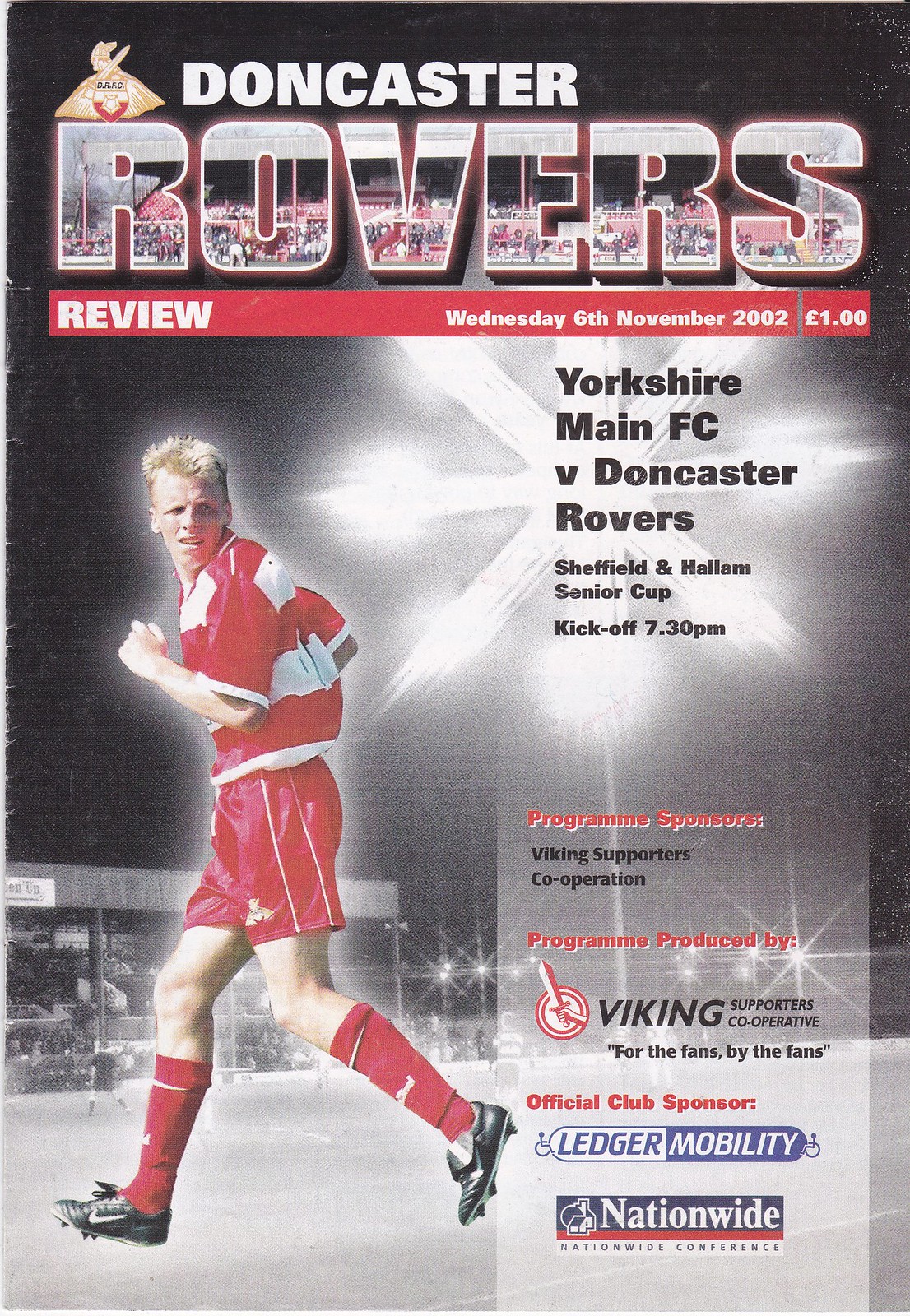This image captures the front cover of a promotional brochure for a soccer event, specifically for the Doncaster Rovers. The bold, dynamic design prominently features a soccer player in action, dressed in a full red kit, including jersey, shorts, and socks, with black cleats. He is depicted running, his face turned over his left shoulder towards the camera. The background is predominantly black but is dramatically illuminated by bright, shining stadium floodlights, creating an intense focal point and a sense of night-time excitement.

At the very top of the flyer, the title "Doncaster Rovers" is displayed in large white letters, with the word "Rovers" featuring a unique overlay of audience members rendered in red. Below the title, a red bar contains white text that reads "Review," followed by the date, "Wednesday 6th November 2002," and the price, "one pound." To the right, further details about the event are noted in black letters, indicating that the game is between "Yorkshire, Maine FC" and "Doncaster Rovers," part of the Sheffield & Hallam Senior Cup, with a kickoff time of 7.30 PM.

Towards the bottom right, several advertisements for event sponsors are neatly arranged. The overall color scheme of the brochure is a striking mix of black, red, white, and occasional touches of blue, enhancing its bold and energetic appeal suitable for a major sporting event.